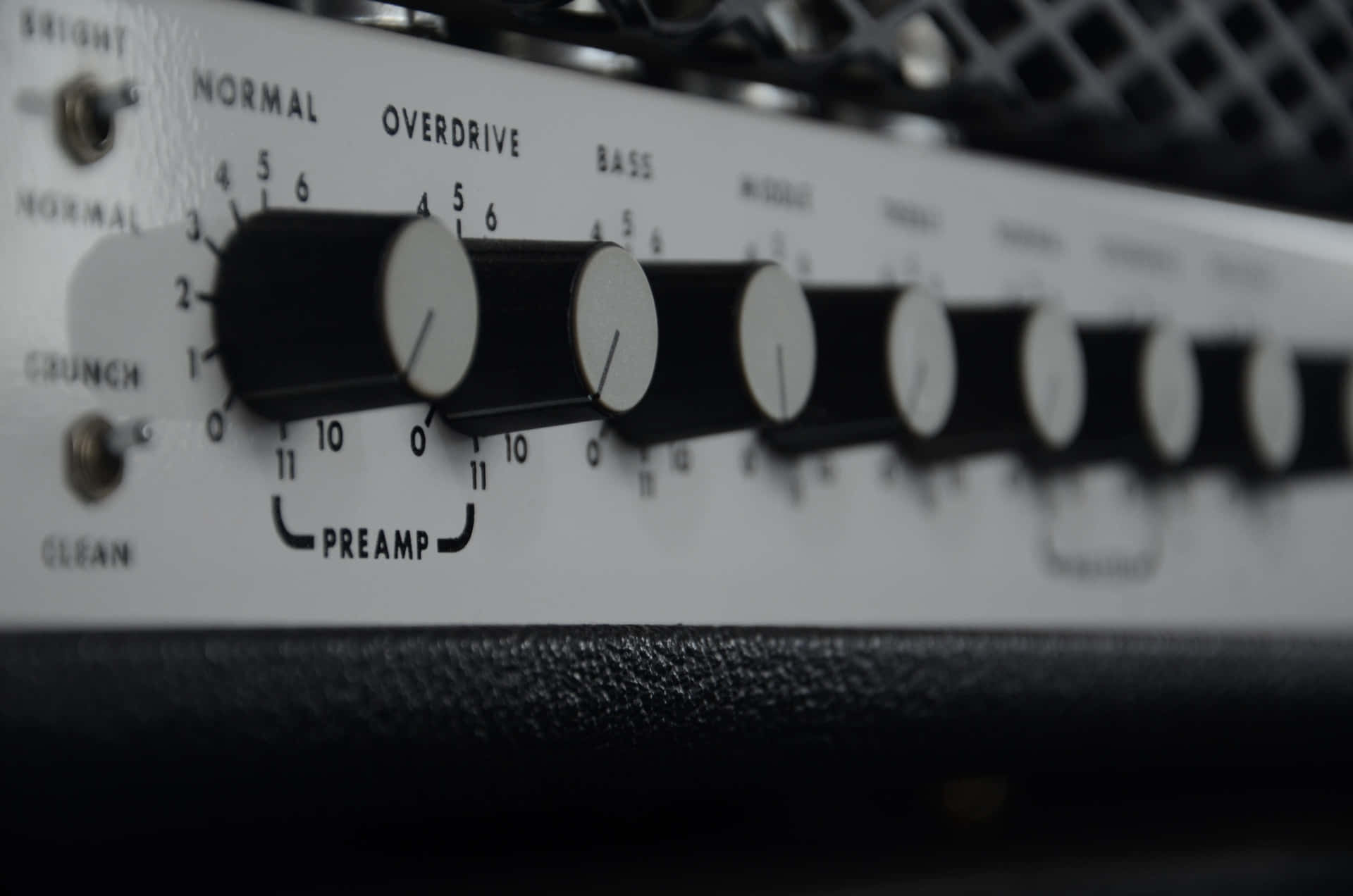This black and white photograph showcases a close-up of a guitar amplifier's control panel. The amplifier features a series of eight finger dials and two switches, all situated on a metal faceplate with black text. The faceplate itself is an off-white color, enhancing the readability of the labels. 

Starting from the left, there are two vertically aligned switches. The first switch, labeled 'Bright' and 'Normal,' is toggled upwards. Below it is another switch labeled 'Crunch' and 'Clean,' which is also toggled upwards. Next to these switches are two dials: the first dial is labeled 'Normal' and is numbered from 0 to 11, currently set at 0; the second dial is labeled 'Overdrive,' also ranging from 0 to 11 and set at 0. Beneath these two dials is a label reading 'Preamp,' connecting the controls together.

Continuing to the right, there is a dial labeled 'Bass,' which similarly ranges from 0 to 11 and is set to 11. As we move further right, the remaining four dials become progressively out of focus, making their labels unreadable, though they also appear to follow the 0 to 11 range. The final dial on the far right is partially cut off in the image.

The surrounding cabinet of the amplifier exhibits a black, leather-like texture, providing a stark contrast to the metal faceplate and controls. Together, these elements create a detailed and functional visual representation of the amplifier's control panel.